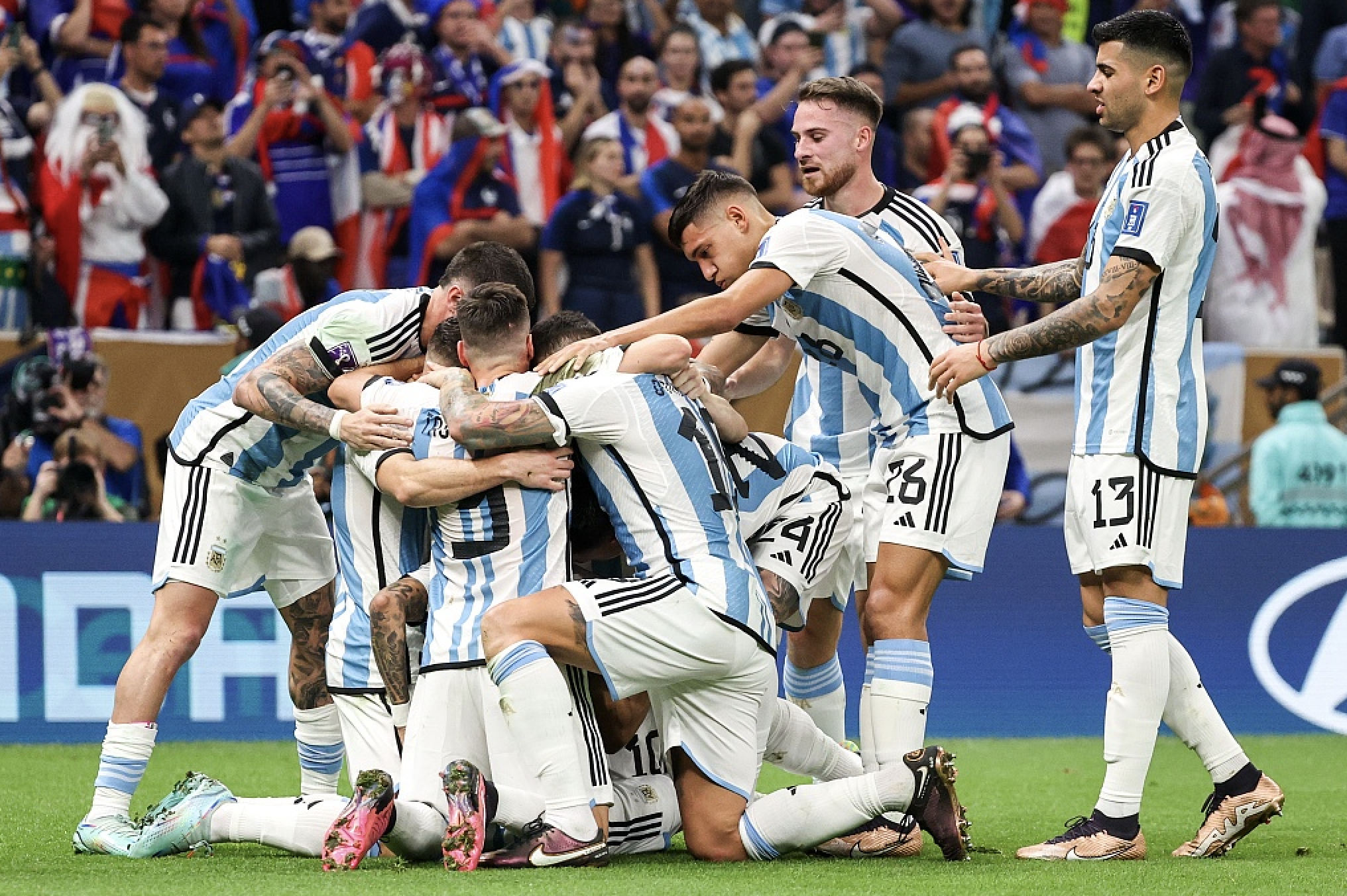In this vibrant and emotional scene captured at the World Cup in Qatar, the victorious moment of Argentina's football team is depicted as they celebrate on a lush green turf field. Central in the image is an exultant Lionel Messi surrounded by his teammates, all adorned in their iconic blue and white jerseys with white shorts, and blue and white socks. Their cleats are visibly dirty, hinting at a hard-fought match. Kneeling and standing, they form a tight-knit huddle, some reaching out and others leaning in, encapsulating the unity and triumph of the moment.

The background reveals stands full of spectators, many clad in the red, white, and blue of the French team, draped in flags and fervently capturing the event on their devices. Visible amongst them are several cameramen and a security guard. A man in traditional Arabic attire stands as a poignant reminder of the host nation's culture. A large blue ball with white letters, presumably saying 'Adidas,' lies towards the bottom of the stands. A sponsor banner with blue and white text adds to the iconic atmosphere of the stadium. The image pulses with the energy of a thrilling match just concluded, celebrating Argentina's momentous victory.